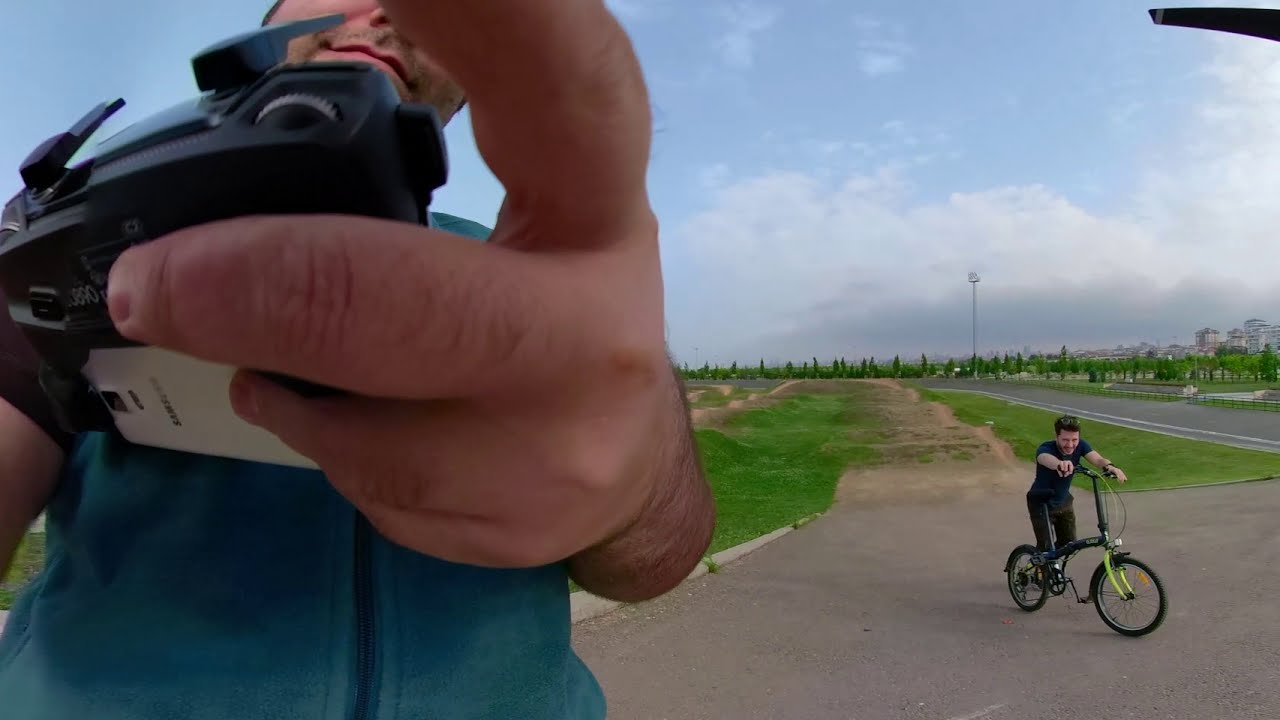In this outdoor photograph, a man is prominently positioned on the left side, holding a black drone controller in his left hand, close to the camera. Details such as the creases and hair on his fingers are visible, as well as part of his face, including his lips, a bit of a mustache, and one nostril. He is dressed in a blue zip-up vest. Behind him, there is a child wearing a blue T-shirt and black pants, riding a bicycle that is blue and lime green. They appear to be on a long, straight paved area adjacent to patches of grass and dirt, resembling a runway. The background features a grassy field, some green patches, trees, a large light pole, and, in the far distance, tall buildings. The sky is expansive, blue with patches of white clouds, contributing to the bright and open atmosphere of the scene. In the upper right corner of the image, the edge of an object, likely the drone responsible for taking the photograph, is visible.